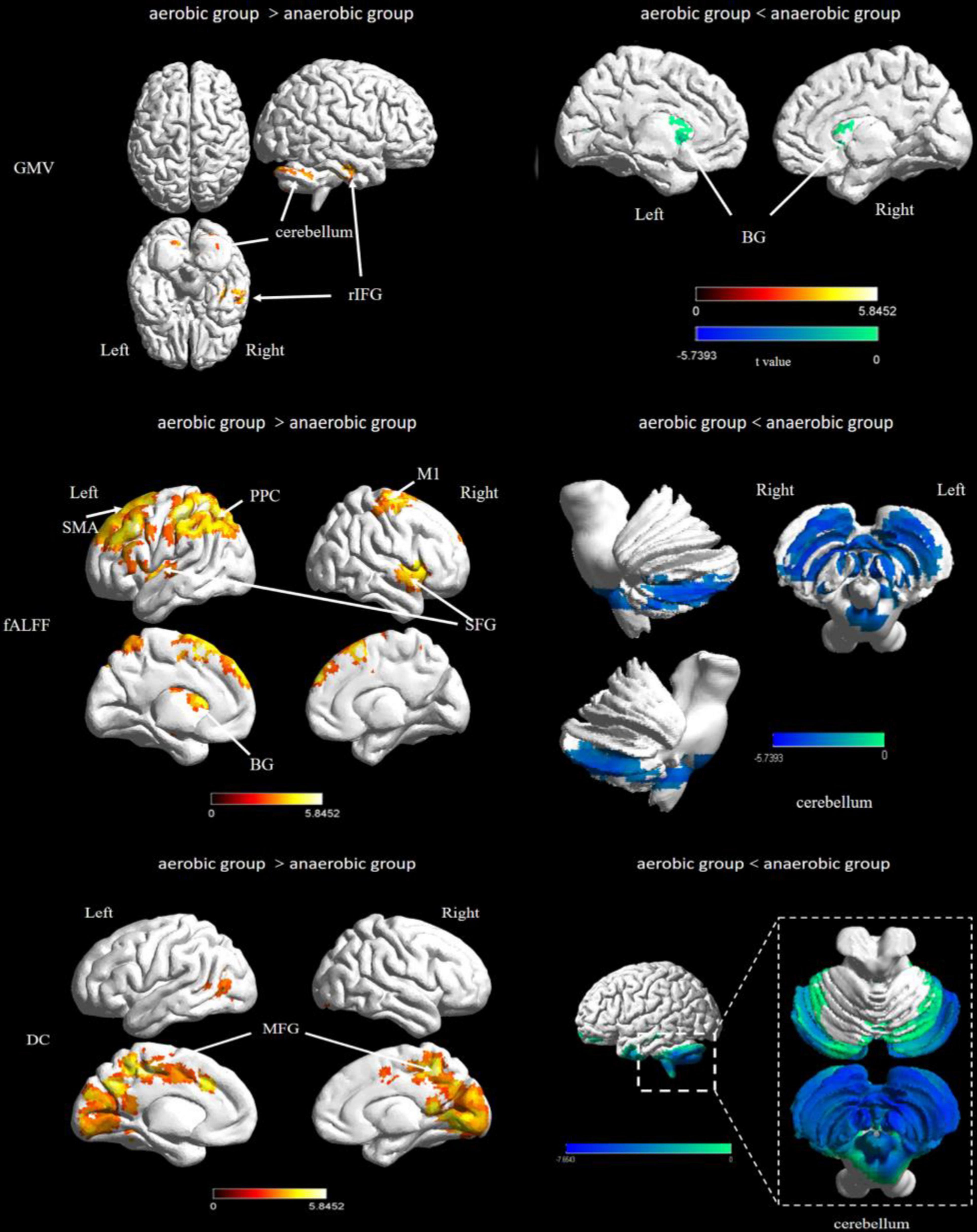This vertically aligned rectangular poster features a solid black background adorned with detailed images of brains viewed from various perspectives. The foreground is occupied predominantly by white illustrations of brains, some accompanied by colorful highlights.

In the top left corner, a cluster of three brain images—displayed from the top, side, and underside views—bear the caption "aerobic group is greater than anaerobic group." These images are marked with smaller white labels, including "left," "right," "GMV," "DRFG," and "cerebellum." To the right, another pair of side-view brain images face each other with a green dot and the label "BG"; a white arrow points to the dot, and the caption reads "aerobic group is less than anaerobic group."

The middle section of the poster features additional brain images. On the left, brains marked with yellow-highlighted areas are labeled "PPC," "SMA," "MI," and "SFG." On the right side, there is an outline resembling a stone bird with feathers, displaying white and blue sections indicating "cerebellum." 

At the bottom of the poster, the corners continue to feature brain imagery with color-coded scales beneath them, predominantly in red, yellow, blue, and green. The bottom right also includes a full brain image and adjacent mysterious geometric figures layered with white, blue, and green.

Throughout the poster, various white text annotations provide additional context, though some of the smaller print details are hard to decipher. Overall, the poster is a rich visual comparison between aerobic and anaerobic brain imagery, enhanced with specific anatomical and functional highlights.